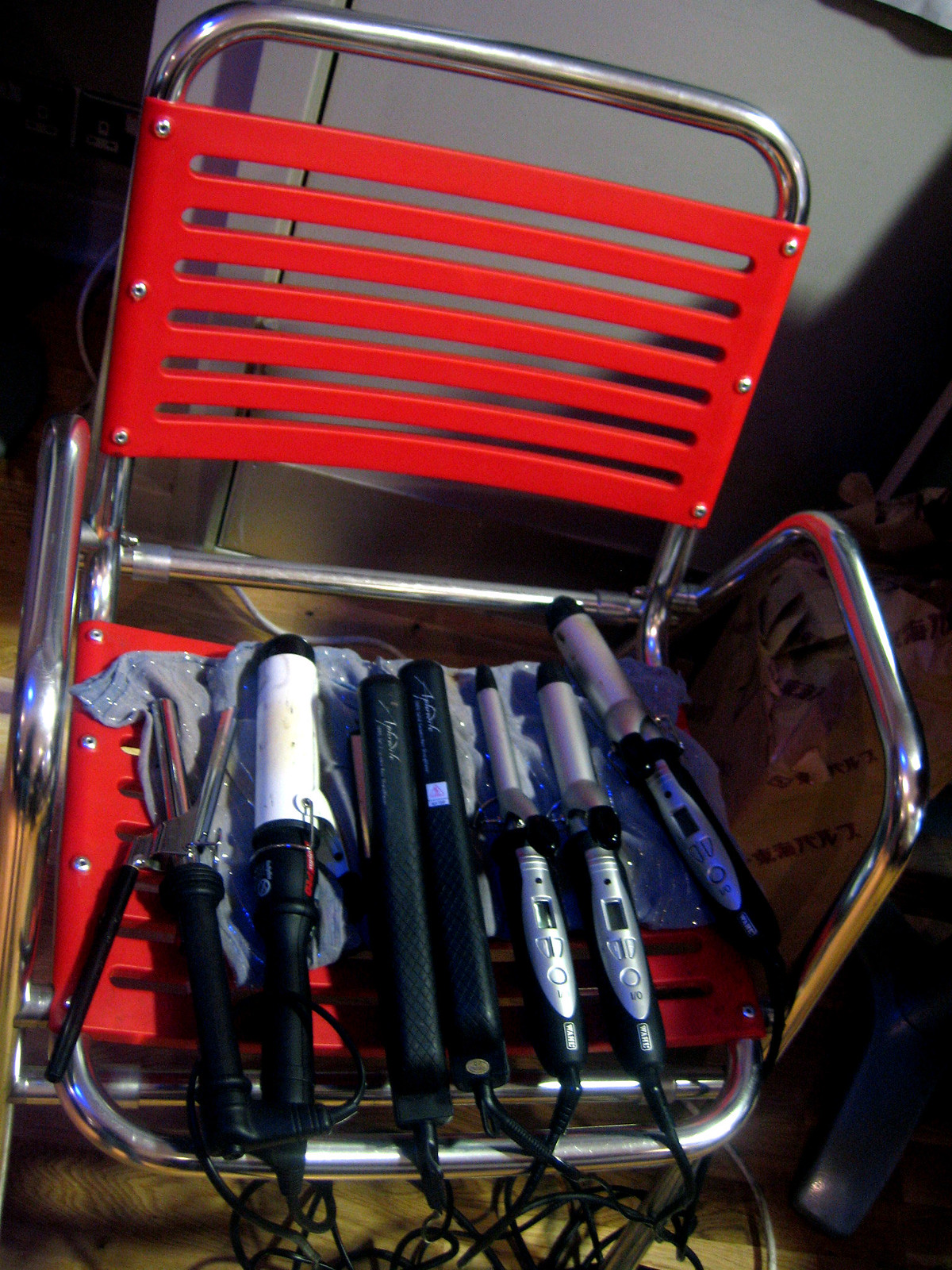This image is of a red plastic and shiny silver metal lawn chair, possibly a folding chair. The chair features shiny silver metal slats and frame, with a reddish plastic seat and backrest. Sitting on the seat of the chair, which is covered by a grayish blue hand towel, are seven hair appliances, including a mix of curling irons and hair straighteners. Most have black handles and gray metal accents around the button areas. Several appliances have unique features, such as silver handles and heating elements, and one has a white heating element with a black handle. The cords from these appliances dangle off the front of the seat, tangled together. In the background, there is clutter on the floor and a white appliance, possibly a washing machine or dryer, adding to the scene.